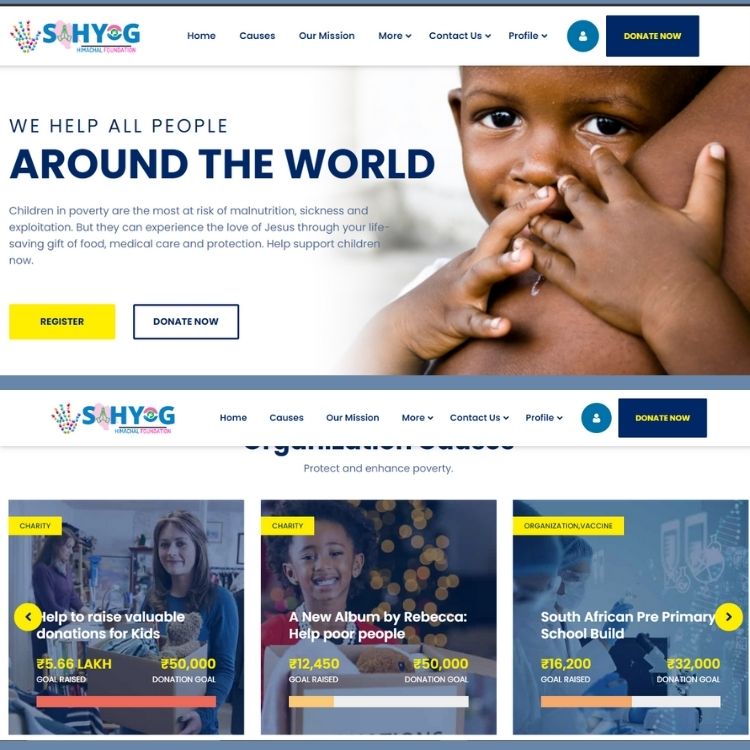This is a detailed caption for the described image:

---

This is a screenshot of a charitable organization's website, potentially named "SIHYOG," though some letters are represented as icons making the exact name unclear. The website's navigation bar at the top right includes links to "Home," "Courses," "Our Mission," with a drop-down menu for "More" and "Contacts," and a "Profile" section with a sub-menu. To the right of these navigational links is a teal circle with a human icon, adjacent to a horizontally elongated rectangle button that reads "Donate Now" in yellow text on a blue background. 

Below the navigation bar is a large horizontal photograph featuring a black child holding onto an adult, possibly the child's mother. The overlaid text states "We Help All People" with "Around the World" in the most prominent font size. Beneath this headline, it reads "Children in Poverty Are the Most at Risk for Malnutrition, Sickness, and Exploitation, but They Can Experience the Love of Jesus Through Your Lifesaving Gift of Food, Medical Care, and Protection. Help Support Children Now." Accompanying this text are two buttons: a yellow "Register" button and a white "Donate" button.

Further down the page, there are three images seemingly part of the same website section, though the continuity isn't entirely clear. The section is titled "Protect and Enhance Poverty." The first image on the left carries the caption "Help to Raise Valuable Donations for Kids" and includes amounts like "5.66 rubles" and "50,000 rubles."

---